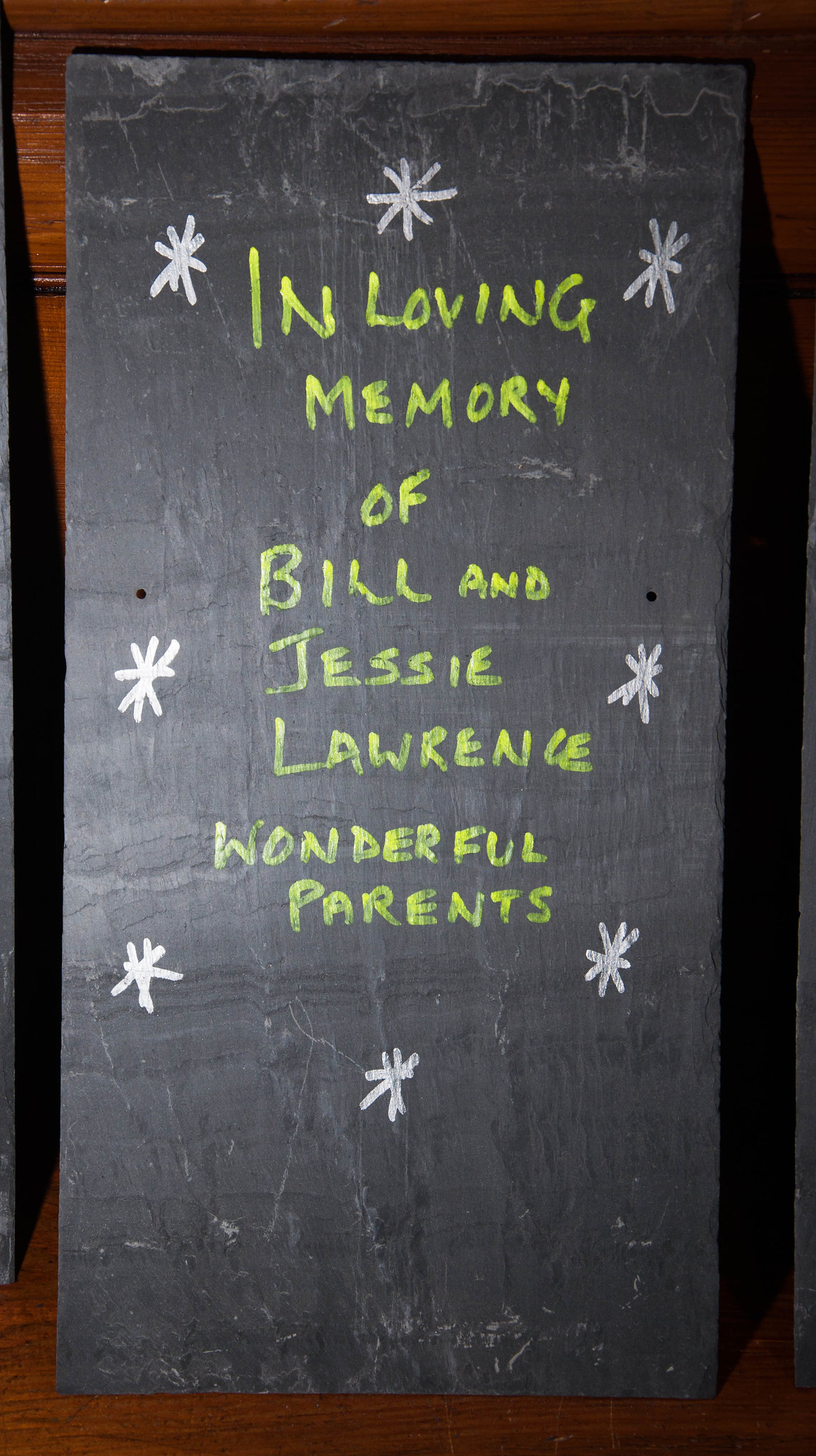This is a photograph of a vertical rectangular blackboard leaning against a wooden wall and resting on a wooden floor. The blackboard is adorned with handwritten text in yellow chalk, memorializing "In Loving Memory Of Bill and Jessie Lawrence, Wonderful Parents," with each word appearing on its own line. The text is framed by white asterisk-like symbols, arranged symmetrically with one at the top middle, one on either side of the text, and several more distributed evenly down the sides, culminating with three at the bottom. These asterisks give the appearance of child-drawn stars or flowers, enhancing the personal and heartfelt nature of the tribute. The setting and presentation suggest a deeply personal and loving memorial from children commemorating their parents.